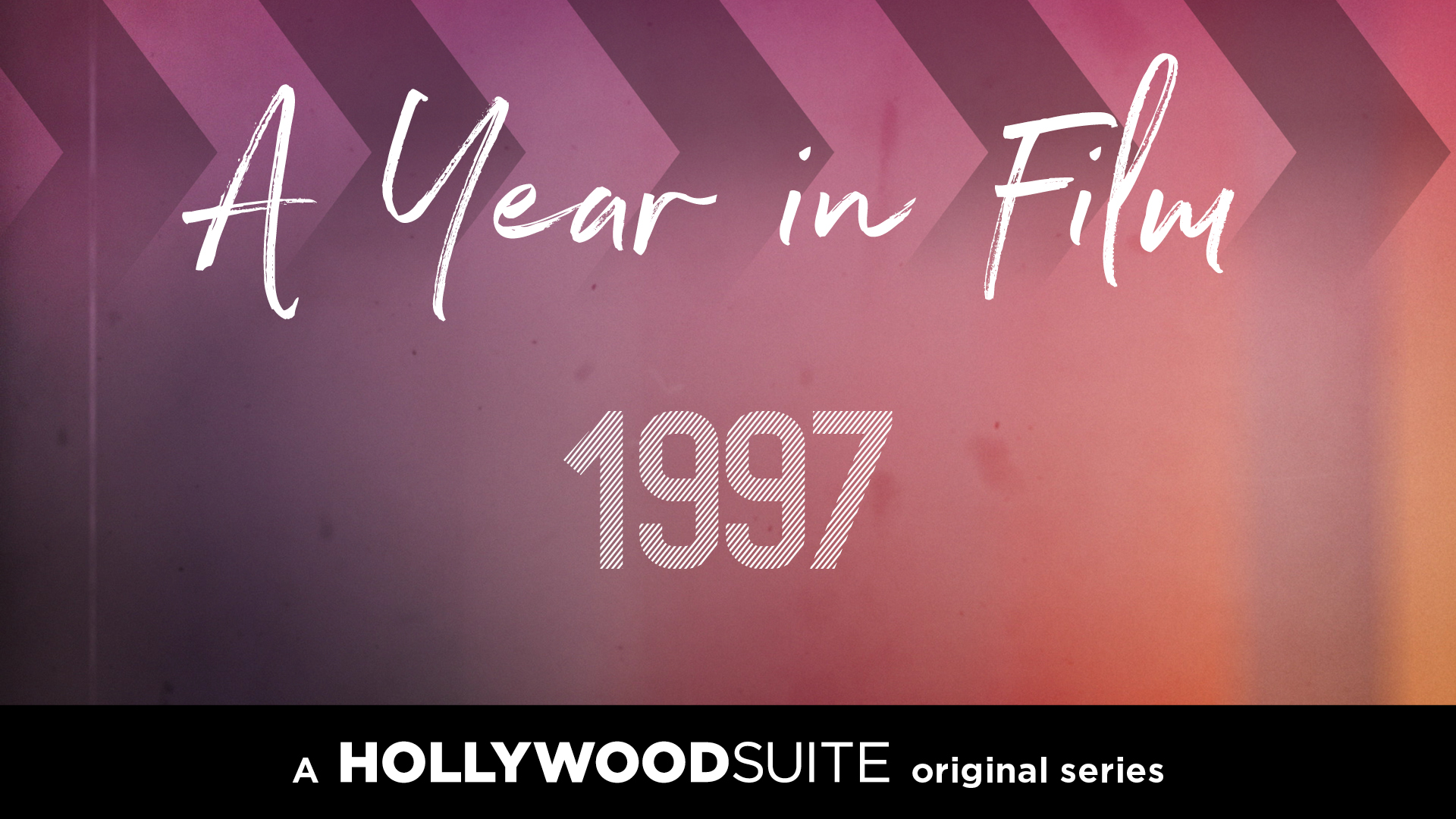The image is a horizontal rectangle resembling a movie poster or advertisement. The backdrop features a dynamic pattern with dark purple zigzag lines interspersed with lighter purple sections, creating an eye-catching effect. Dominating the top portion of the image are five purple arrows pointing to the right. Centered prominently in white handwriting-style text is the phrase "A Year in Film," and directly below this, in gray lettering, is the year "1997" adorned with diagonal black stripes. The bottom section of the image is a horizontal black banner, which bears the inscription "A Hollywood Suite Original Series" in crisp white lettering, tying the entire composition together.